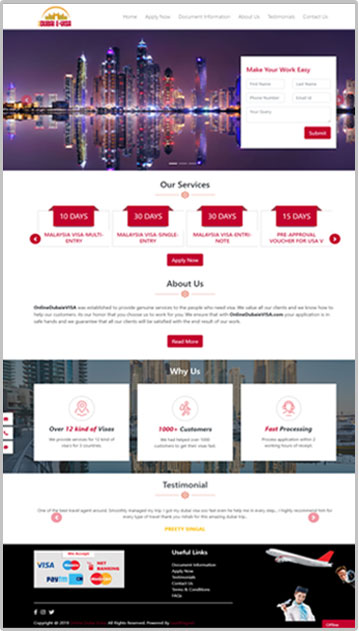**Descriptive Caption:**

This image is a low-quality screenshot of a travel website. The upper section features a white banner with a series of navigation tabs. To the upper left, there's a logo and the website's name. Below the banner, there's a striking photograph of a city's skyline at night, showcasing illuminated skyscrapers reflecting off the water.

On the right side of the photograph, a white box houses various clickable buttons with the text "Make Your Work Envy" displayed prominently in red. A red button is positioned at the bottom right corner of this box.

Further down, a section marked "Our Services" appears against a white background, displaying four small, red house-like icons, each with a different number, possibly indicating stay durations (e.g., 30, 10, 15 days). Each icon is accompanied by some illegible red text. The section includes arrow symbols on both sides for navigation and a red button beneath it.

The "About Us" section follows, featuring a brief paragraph of text and another red button. Below, the "Why Us" section has a daytime city skyline background and includes three informational boxes, each with its own icon, though the text is unreadable.

The "Testimonial" section comes next, containing a sentence or two with arrows for scrolling through additional testimonials. At the bottom, a box lists various accepted payment methods and provides extra information alongside "Useful Links." In the bottom right corner, there's a graphic depicting a plane and a woman.